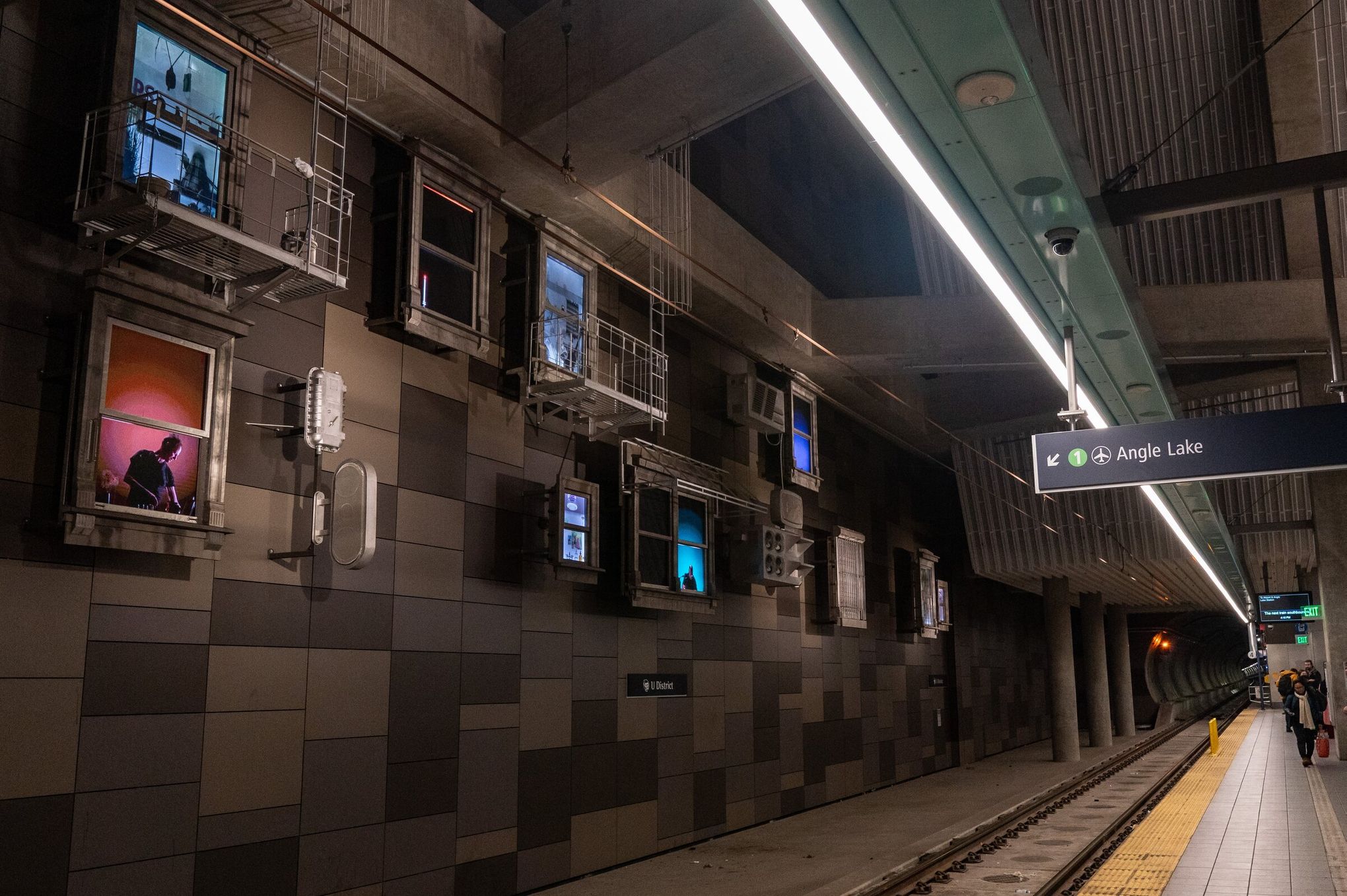The photograph depicts a bustling subway station named "Angle Lake," evident from the overhead sign featuring an airplane icon and the number 1. Situated on the opposite side of the tracks, the wall showcases a series of illuminated screens designed to mimic apartment windows, adorned with vibrant hues. These faux windows are set against a patchwork of colorful bricks, in shades of dark brown, light brown, and purplish brown. One screen notably displays a DJ bathed in a reddish-pink glow, while another presents random artifacts in bluish tones, suggesting a digital installation rather than real windows. The station platform, marked with a distinct yellow safety line, accommodates a few commuters waiting for the next train. The ambiance is further enriched by an orange light flickering deeper into the tunnel and signage that evokes the feeling of an airport terminal. Casual travelers, dressed in everyday attire, prepare to board as exit signs provide clear guidance for egress.